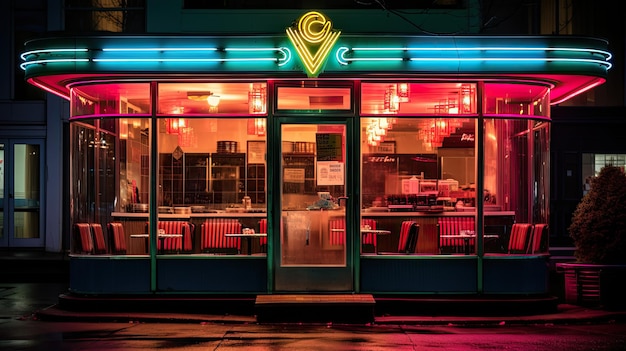This photo depicts an old-school diner taken from the outside at night. The establishment features predominantly glass windows, offering a clear view inside. The interior is illuminated with a range of bright pink lighting, and there are chandeliers hanging from the blue ceiling. The diner is empty with no people inside or staff visible. The seating consists of red and black booths, and there are numerous tables arranged for dining.

Prominently displayed atop the diner are neon signs: the letters "C" and "B" in yellow, complemented by blue and green neon lines along the edge of the roof. A V-shaped yellow neon sign is centralized above the establishment, and a green-framed glass door serves as the main entrance. Outside, there's a tree to the right and a white building adjoins the diner on the left. Potted shrubs add a touch of greenery to the exterior.

The scene is bright and inviting, projecting an atmosphere that looks fantastic and suggests the diner is a great place for a meal despite appearing closed at the moment.